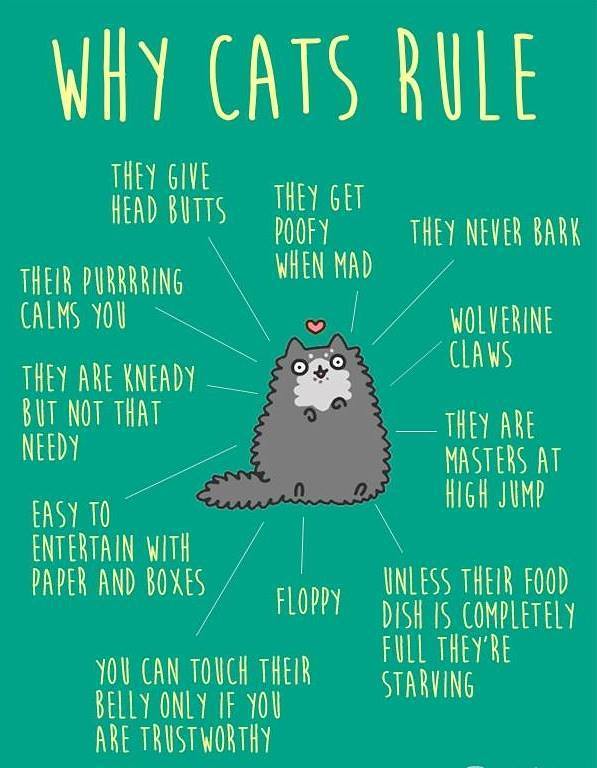The image is a humorous and colorful infographic with a blue-green background, featuring a simple yet adorable illustration of a gray and white cat at its center. A red heart hovers above the cat's head, enhancing its cute appeal. The title "Why Cats Rule" is displayed prominently at the top in bright yellow text. Around the cat, at multiple levels, there are various bullet points connected by white lines, each highlighting endearing and quirky cat behaviors. These points include: "They Give Head Butts," "They Get Poofy When Mad," "They Never Bark," "Wolverine Claws," "They Are Masters At High Jump," "Unless Their Food Dish Is Completely Full, They're Starving," "Floppy," "You Can Touch Their Belly Only If You Are Trustworthy," "Easy To Entertain With Paper And Boxes," "They Are Needy But Not That Needy," "They Are Needy (like kneading bread)," and "Their Purring Calms You." The overall style suggests that it could be a poster or comic, and the layout efficiently showcases why cats are adored by many.